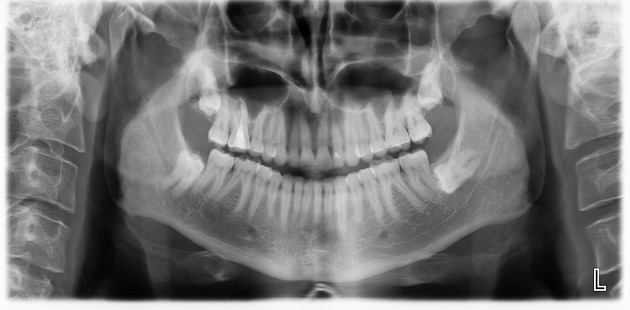This black-and-white x-ray image predominantly features a detailed view of a skull, likely from a gorilla, given the larger nostrils compared to a human and the overall structure. The image captures both the top and bottom rows of teeth, which bear a resemblance to human teeth but are somewhat thinner. The skull is the primary focus, zoomed in to highlight the orbital eye sockets and dental arrangement. Flanking the central skull on both sides are the individual bones of the arms, and there are vertebrae visible, suggesting this is more than just a typical skull x-ray. Though slightly blurred in the background, the bones create a symmetrical outline around the skull. Additionally, there's a distinct white letter "L" on the bottom right corner of the image, possibly indicating positioning or orientation in the x-ray.